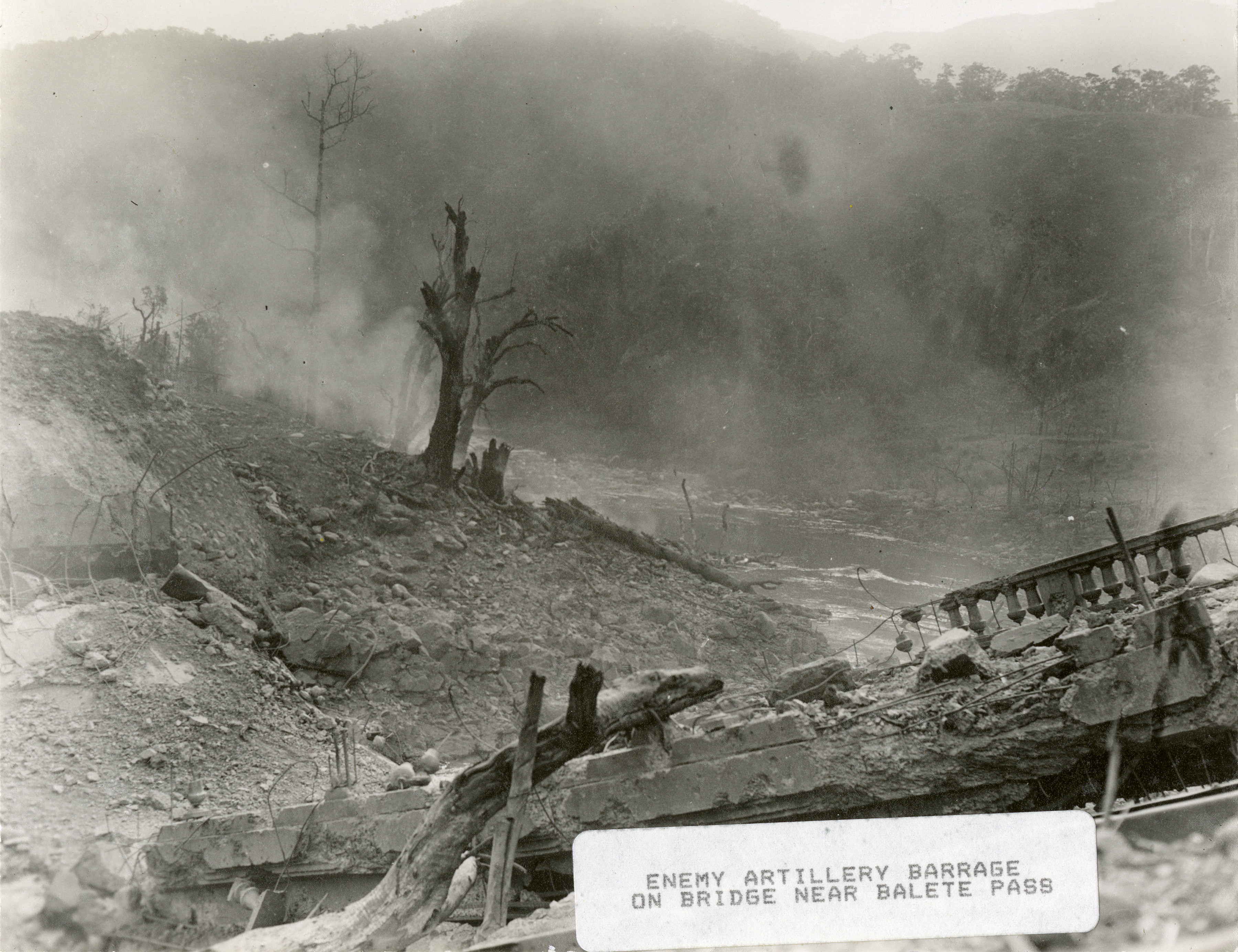This vintage black and white photograph captures a bleak, war-torn scene of devastation, identified by a stamped caption at the bottom as an "enemy artillery barrage on bridge near Balet Pass." The image likely dates back to World War II and is set near Balet Pass, a significant location in the Philippines during the conflict. The foreground is dominated by a chaotic spread of rubble and rocks where the destroyed bridge once connected to the land, flanked by the remains of dead, limbless trees. Smoke lingers over the decimated landscape, adding to the somber atmosphere. In the background, the ruins give way to a serene but stark contrast of undamaged trees, rolling hills, and a river, underscoring the intrusive violence of war amidst nature's calm persistence. The absence of people and structures enhances the desolation and magnitude of the destruction depicted.